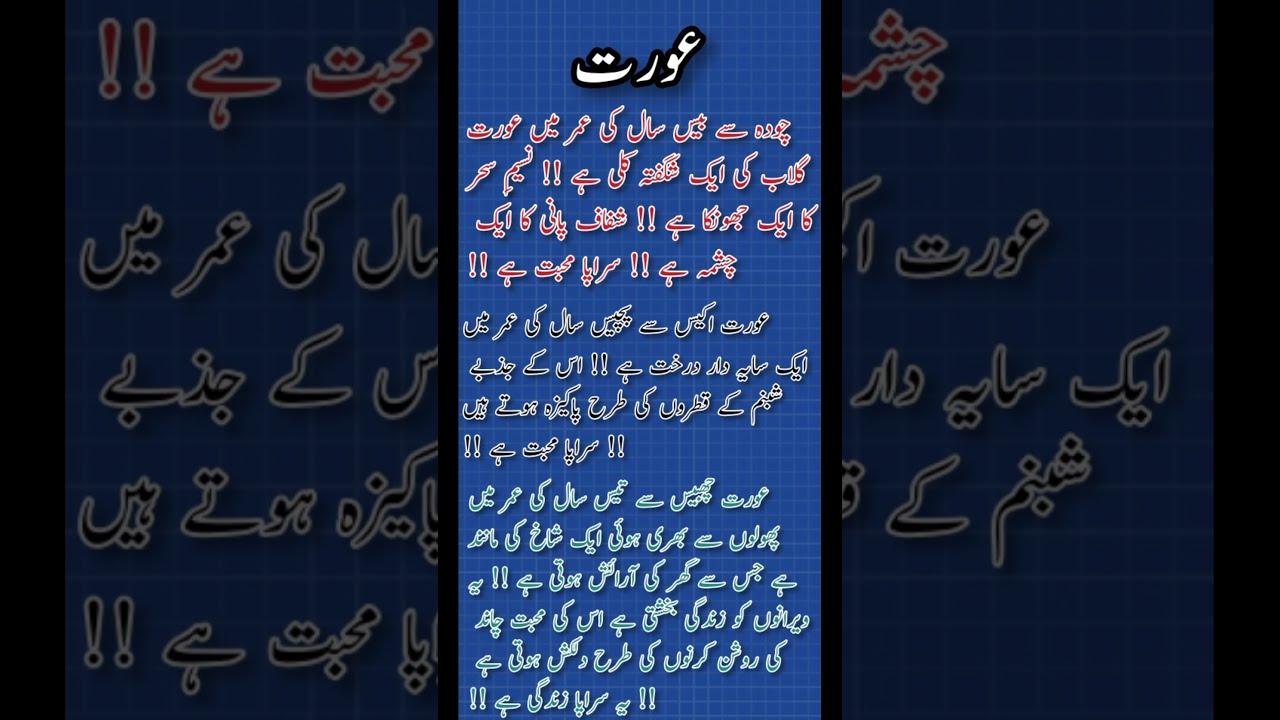The image consists of three vertical panels, with the central panel serving as the main focus. The background is predominantly blue with a grid of white lines reminiscent of graph paper. Centered within this main panel is a vertical, lighter blue rectangle featuring foreign symbols or characters that do not resemble the Japanese, Chinese, or the English 26-letter alphabet. At the top of this central vertical panel, there are three white symbols bordered in black. 

The writing on this central panel is divided into multiple sections and colors: four lines of pink characters, followed by four lines of black characters, each highlighted with white borders, and finally, approximately six lines of green characters. Surrounding the central area, the right and left thirds of the overall image display additional sections of the main vertical panel, effectively splitting it into three parts.

In addition to the central symbols and script, there's a notable face-like figure at the top that somewhat resembles a frog with a limb or hand reaching upwards. The primary colors used in the image are blue, white, and black, with additional accents of pink, red, and green characters. Notably, there are no numbers or other text within the image.